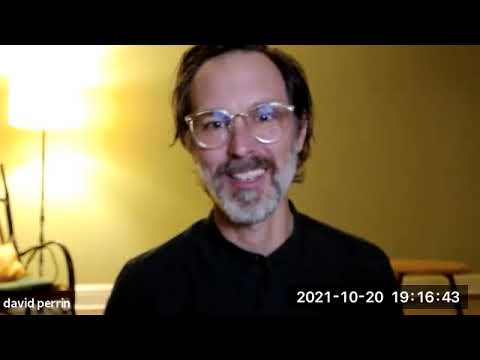The image is a low-quality, blurry screen capture, possibly from a video call, showing an older white man in his late 60s named David Caron. He has short black hair with a receding hairline, balding at the top, and some length at the back. His hair is parted on the right side, drooping slightly to the left. He wears prescription glasses with light-shaded lenses and has a full beard and mustache that are predominantly white and black with very little brown remaining. 

David is dressed in a black top and is seated in a room with an orange background, which features a light and a chair on the left side and a stool on the bottom right. The bottom right corner displays a timestamp in white text that reads "2021-10-20 19:16:43." Additionally, there are black borders on the top and bottom of the image, and the name "David Caron" appears in white text on the bottom left.